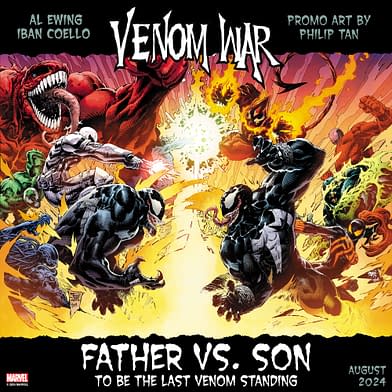This image appears to be a highly detailed and dramatic cover for a Marvel comic book or magazine titled "Venom War," slated for release in August 2024. The text prominently features the names of the authors Al Ewing and Ivan Coelho, with the promo art credited to Philip Tan. The central theme is a confrontation between two characters, identified as father and son, with the caption, "Father vs. Son to be the last Venom standing."

In the foreground, two muscular Venom characters are locked in a fierce battle amidst a storm of fiery explosions and swirling energy, depicted in intense yellow and orange hues. Surrounding them are various monstrous figures, colored in shades of green, red, and silver, adding to the chaos and drama of the scene. The overall aesthetic is dark and gripping, with a black background and predominantly white text that contrasts sharply with the vivid colors of the artwork. The style and presentation suggest a dynamic and action-packed storyline, characteristic of Marvel's dramatic comic book covers.